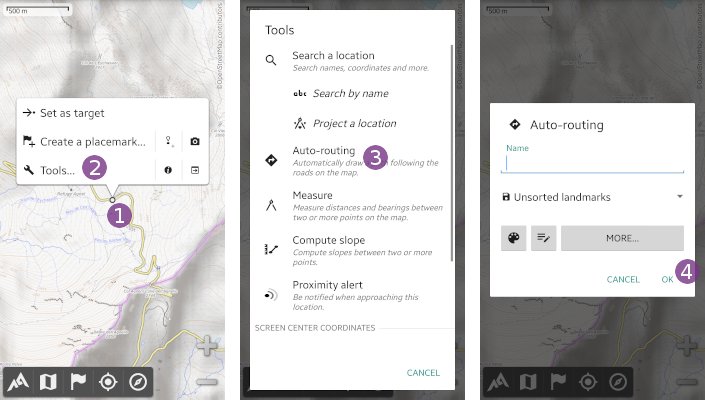This is a set of three images depicting a navigational application interface, showcasing a sequence of actions to set up a route.

1. **First Image (Left Panel)**: The interface displays a map with two prominent purple circles. An arrow labeled "Set as target" points to one of the circles. Below the map, several interactive icons are visible:
   - A flag with a plus sign labeled "Create a placemark."
   - An exclamation mark icon.
   - A camera icon.
   - A tools icon, labeled "Tools," underneath the flag icon.
   - A purple “2” above a pop-up box with the number “1.”
   
2. **Second Image (Middle Panel)**: This screen expands on the "Tools" section. The header reads "Tools," followed by instructions:
   - "Search your location. Search names and coordinates and more."
   - The interface shows two clickable locations, each marked by a blue dot. The first blue dot is selected initially.
   - Another blue dot is shown which, upon clicking, indicates the selection of the "Tools" option, consistent with the instruction to "Search a location. Search by name, project location."
   - Below, an option labeled "Auto-routing" is present, marked by a purple circle with a white number “3.”

3. **Third Image (Right Panel)**: This screen focuses on the "Auto-routing" process.
   - The header reads "Auto-routing."
   - There is a text field labeled "Name" for inputting the route name.
   - Towards the bottom, a purple circle with a white number “4” is associated with an "OK" button, indicating the final step to confirm and set the auto-routing.

This sequence of images guides the user through selecting a target, accessing navigation tools, and setting up an auto-route within the application.